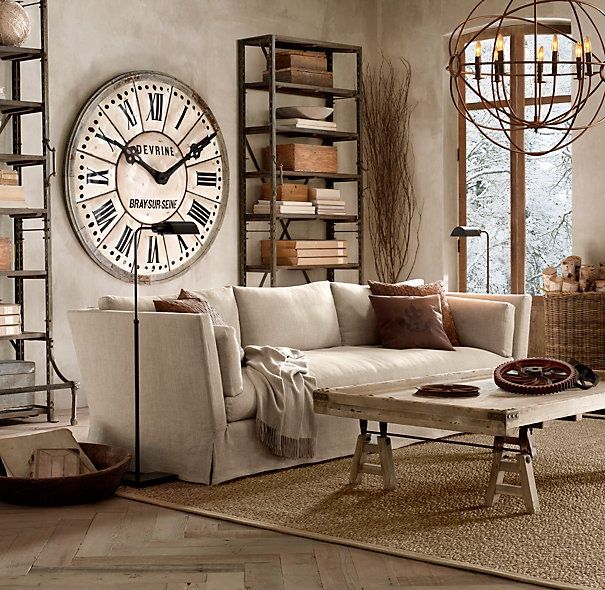This photograph showcases a sophisticated and modern living room dominated by shades of beige, accented by darker brown and black trims. The room features a central off-white couch adorned with three brown pillows and a matching beige throw blanket draped over its side. Positioned against the wall, the couch is framed by an oversized clock with Roman numerals and black hands hanging above it. Flanking the couch on both sides are matching metal bookshelves in dark polished brown, filled with various brown and white objects. A light beige wooden table with intricate legs stands on a large tan rug, with decorative brown wheels placed atop it. Adjacent to the couch are two black lampposts; the one on the left side accompanies a wooden bucket with light beige books, while the one on the right side is accompanied by a wicker basket containing wood logs. Large floor-to-ceiling windows on the right-hand side of the living room reveal a snowy outdoor scene, adding to the room's serene ambiance. The chevron-patterned wooden floor ties the entire look together, completing this stylish and cohesive interior setting.